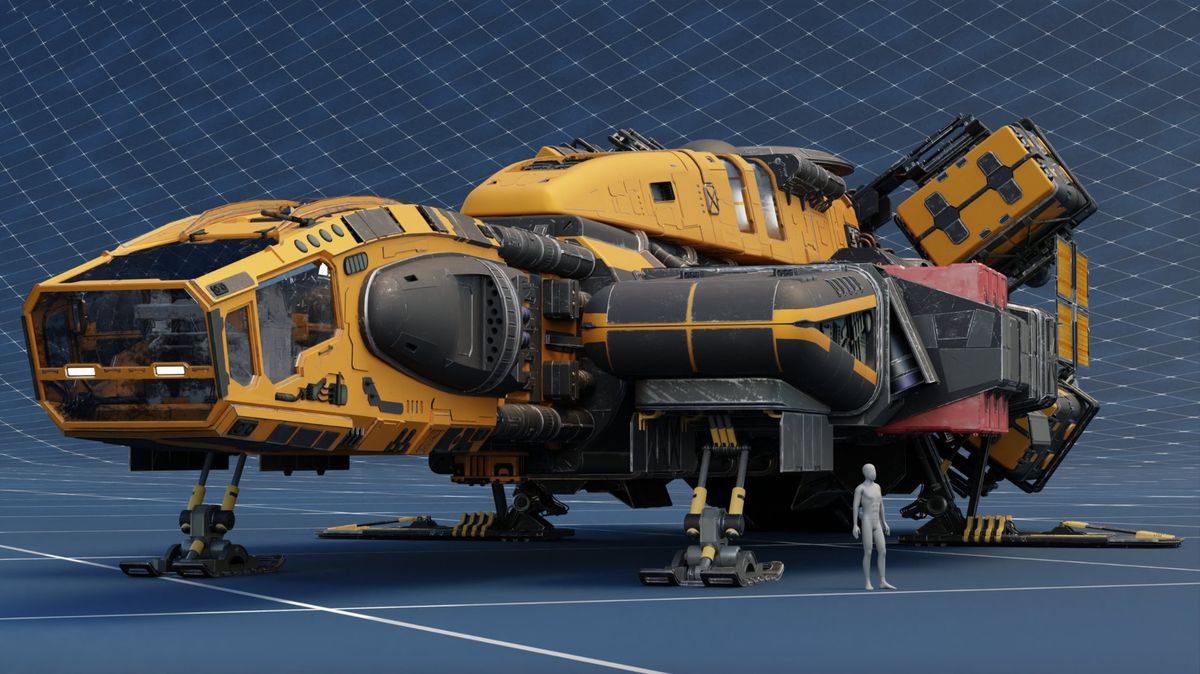The image depicts a computer-animated scene featuring a colossal yellow, black, and red spaceship, supported by at least four landing legs and adorned with large windows and a box-shaped pilot's cabin made of clear glass. It is set on a navy-blue grid-marked surface, with light gray grid marks extending onto the navy-blue ceiling above. An unclothed, hairless, gray robot-like figure or mannequin stands at the base of the spacecraft, towards its right side, serving as a scale reference against the enormous structure. The spacecraft features white headlights on its left side and appears to be situated in an industrial or construction-like environment, without any visible passengers or pilots.